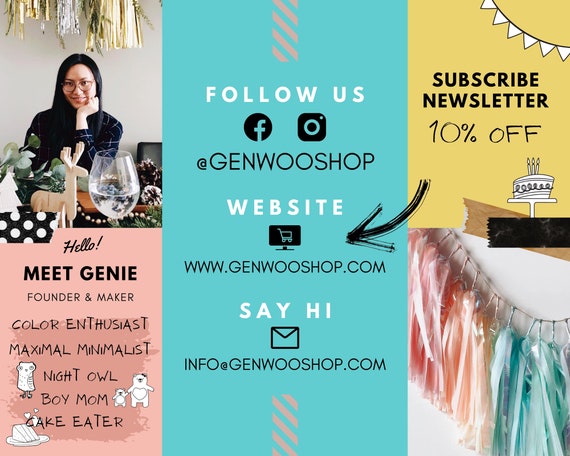The image is a three-part promotional graphic for a business named Jin Wu Shop. 

The leftmost section features a woman of Asian descent, likely Jeannie, sitting at a decorated table that includes a wooden moose figurine, a large wine glass, and some botanical elements. Behind her, there's a gold fringed banner. A pink caption below her introduces her as "Jeannie, founder and maker, color enthusiast, maximal minimalist, night owl, boy mom, cake eater," with small graphical representations like a white cake and teddy bear.

The middle section has a light turquoise background featuring the text "Follow Us" in white at the top. Below it are black Facebook and Instagram logos alongside the handle @JinWooShop. A black arrow points to an illustration of a computer screen with a shopping cart. Below that, the website www.JinWooShop.com is listed, and further down, it says "Say hi" in white next to an envelope icon, followed by the contact email info@JinWooShop.com.

The rightmost section bears a yellow background calling for newsletter subscriptions, with a promise of 10% off. Below this text, there is an illustration of a white cake on decorative tape. At the bottom, a pastel-colored fringed banner adds an extra festive touch, reminiscent of intricate table decorations found at banquets.

This cohesive blend of elements highlights Jeannie's unique personality and her vibrant business, making an engaging and inviting impression.